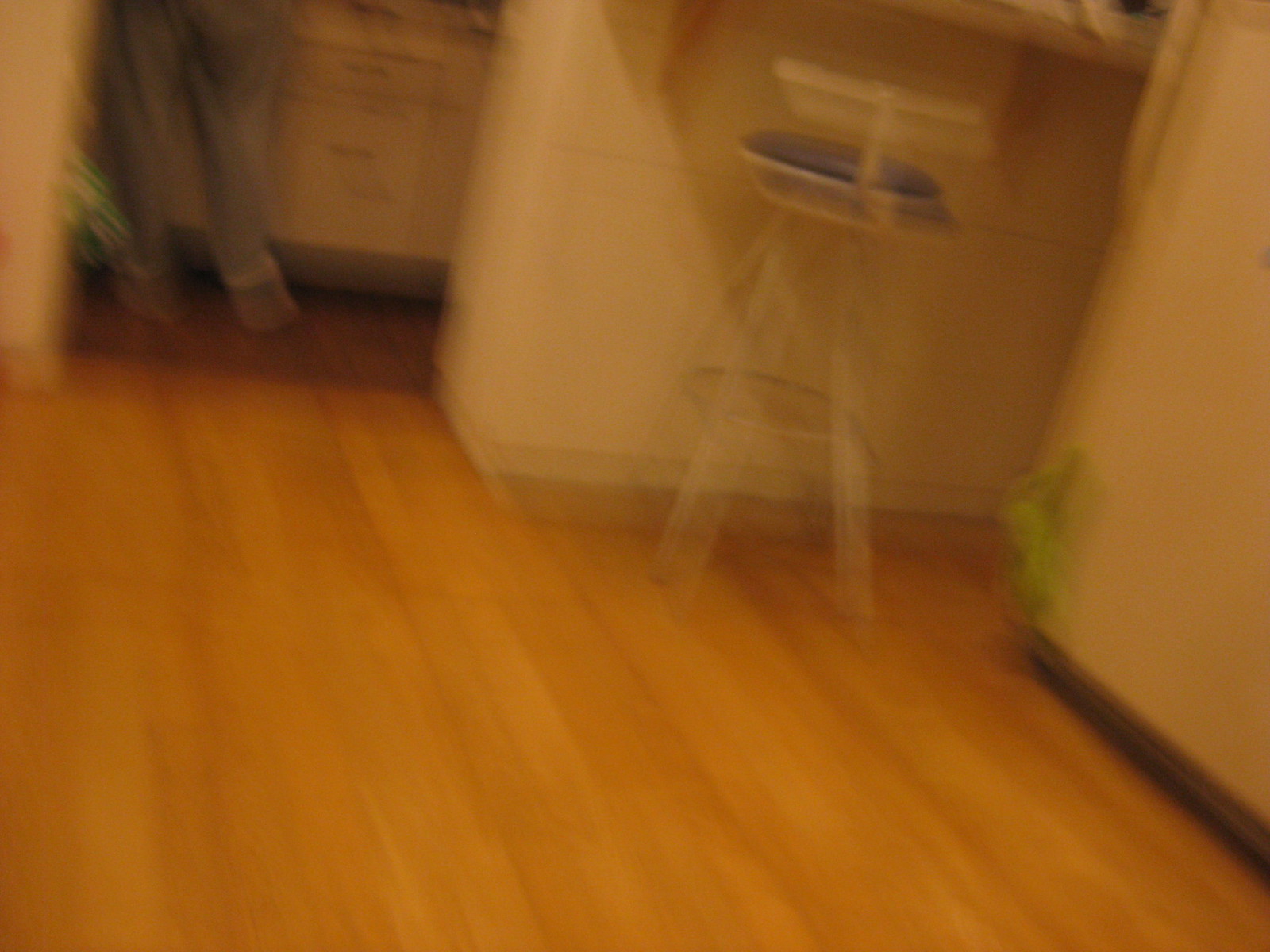The image is quite blurry, making it difficult to precisely identify the location, though it vaguely resembles a doctor's office. The setting features a light wood floor paired with either gray or brown molding along the edges. Central to the image is a white wire stool with a blue seat, positioned in front of what could be a desk or counter. In the background, white wooden cabinets are visible. The lower half of a person, dressed in blue jeans and brownish socks, can be seen near the cabinets.